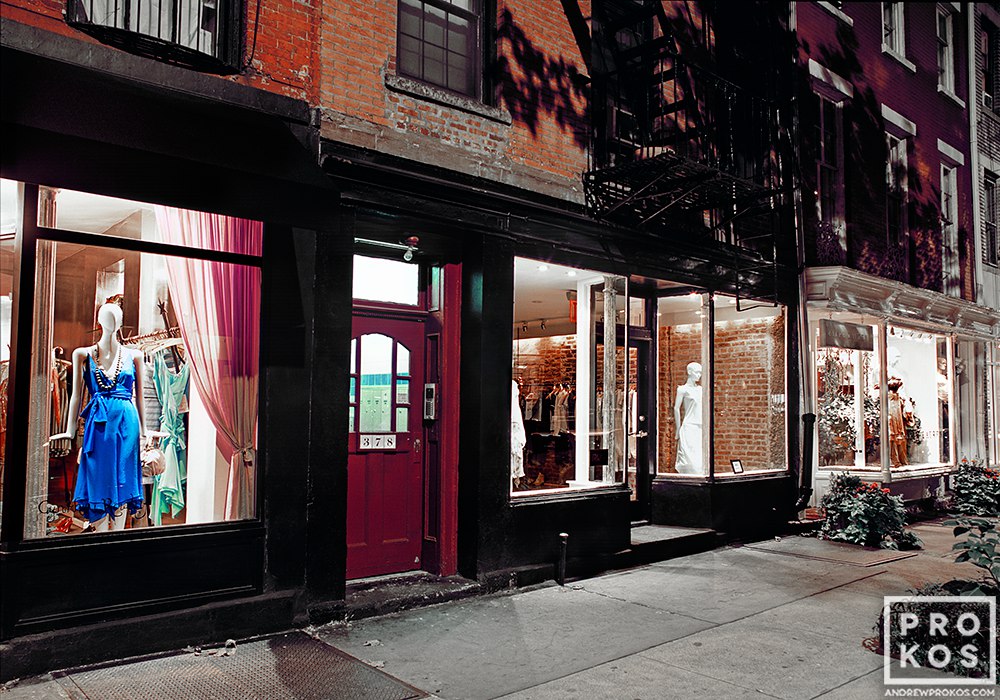The image portrays a nighttime city street scene with a row of very old, brick storefront buildings, which appear to be in New York City. The centrally located older buildings are constructed from brick and feature painted black wooden exteriors. Each of the storefronts showcases dressmaker's dummies adorned in various dresses. The first mannequin displays a blue dress with beads, complemented by purple to tan curtains on the left side. To the far right, another mannequin features a white dress. The address "378" is visible on a maroon door, suggesting an entryway to one of the shops or apartments situated above the stores. Notably, the name "Prokos" and the website "andrewprokos.com" are inscribed in the bottom right corner of the photograph. The diverse color palette in the image includes hues of red, orange, blue, green, beige, brown, black, white, tan, magenta, and pink, adding vibrancy to this vintage cityscape. Fire escapes and older windows further accentuate the historical charm of the scene.